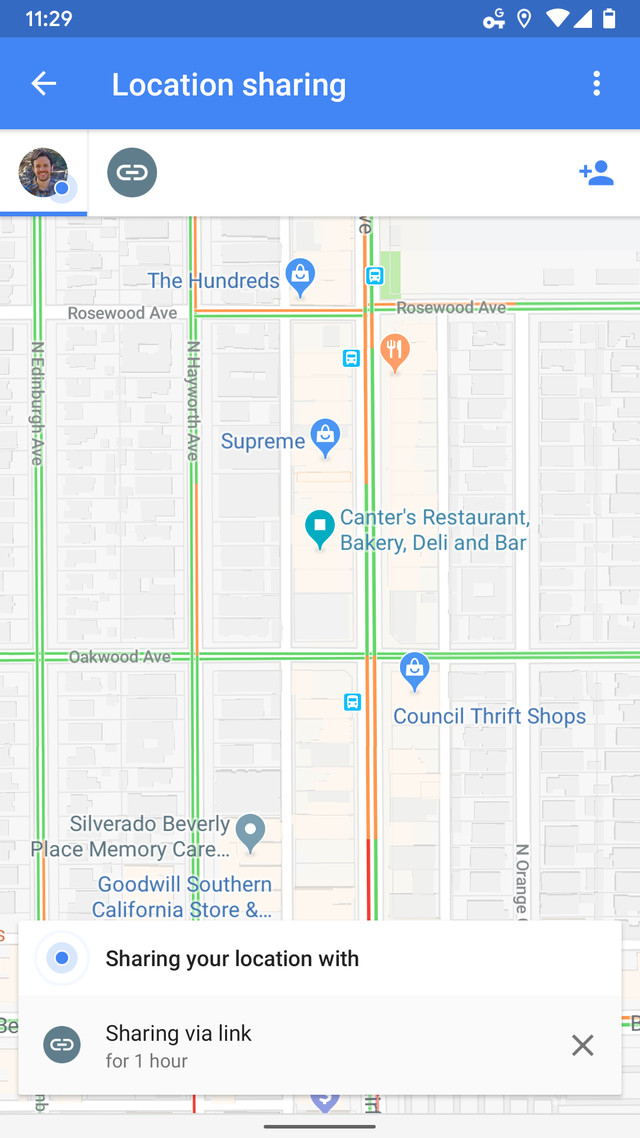A detailed screenshot of a smartphone display showcases various elements. In the top left corner, in white text on a blue background, it reads “11:29.” Icons such as a key, Google “G,” pen, Wi-Fi, battery, and signal strength are also featured, all in white on the same blue background. Below, in white on blue, it says “Location sharing” next to three vertical dots and a left-pointing arrow. 

The next section shows a user profile indicated by a solid blue dot, adjacent to a grey circle with a link icon, and a solid person icon typically used for adding contacts. 

The main section of the screenshot is a detailed map prominently marking a location called "The Hundreds." It highlights surrounding roadways with lines indicating traffic conditions: green for smooth traffic and red for congestion. Nearby landmarks such as "Supreme" and "Cantor's Bakery" are visible, along with "Council Thrift Shops." A circle highlights the user’s current location, indicating it is being shared. 

At the bottom of the screen is a pop-up bar, providing the option to share your location, featuring an "X" inside a small white box, and a grey box beneath it. The image effectively conveys the functionality of a location-sharing feature in a mapping application.